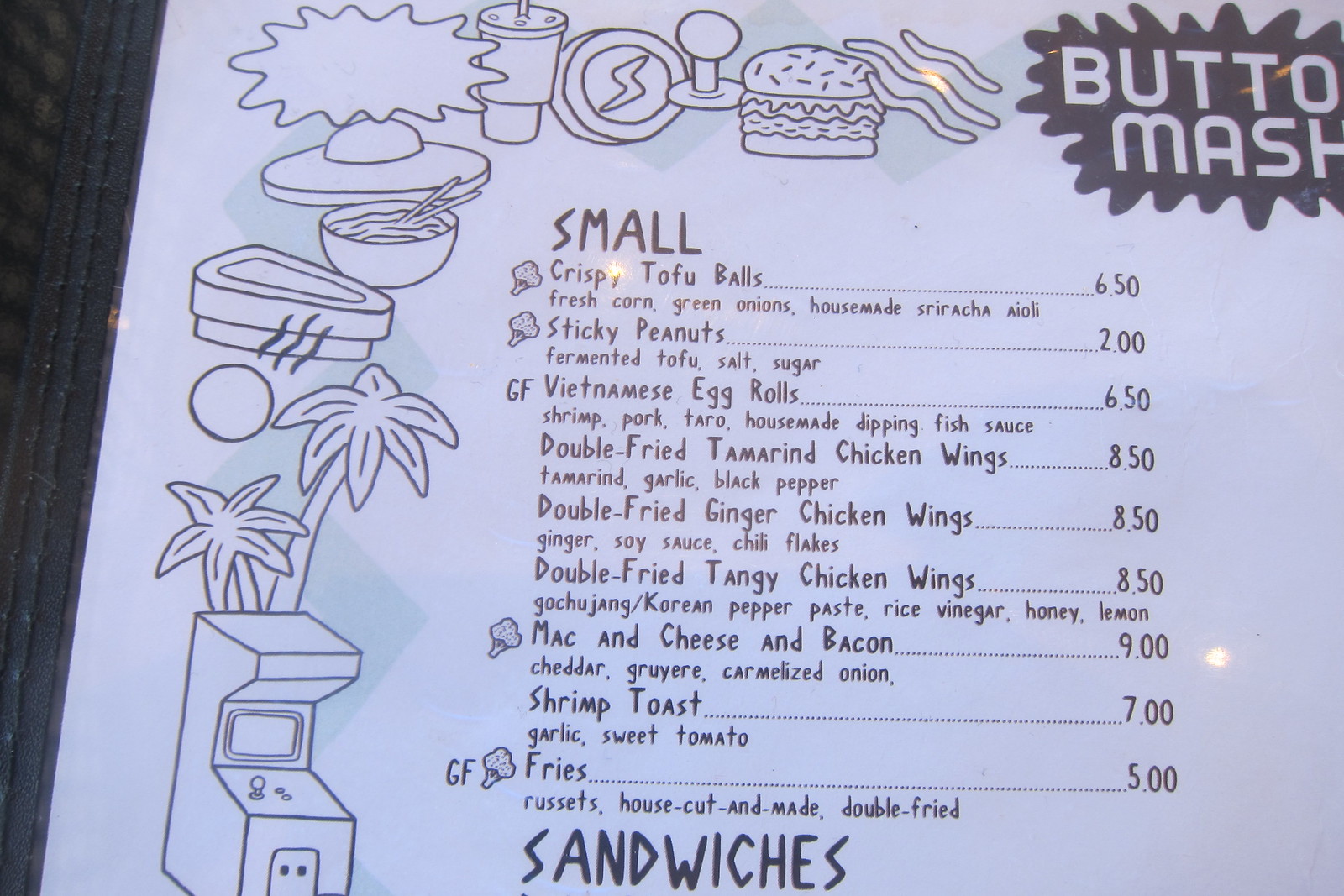A detailed fragment of the Buto Mash restaurant menu captures attention with its eclectic design and diverse offerings. The top portion of the menu features vibrant images of a soda container, a hamburger, and a serving of fries, tantalizingly indicative of the hearty meals on offer. Along the side, whimsical illustrations such as spaceships, a Thai noodle dish, and a video game create a playful and engaging atmosphere.

The menu categorizes some items under the "Small" section, highlighting crispy tofu balls, sticky peanuts, Vietnamese egg rolls, mac and cheese with bacon, and fries. These small delights promise a variety of flavors, from the fusion of Vietnamese cuisine to comforting American classics. 

Beneath the "Small" section, the menu lists sandwiches, although this part appears to be cut off, hinting at an extended list of delicious options awaiting discovery. The visual appeal combined with the menu's content suggests Buto Mash is a fun and inviting place to dine, with affordable prices ranging from $2 for sticky peanuts to around $9. The thoughtfully designed layout features item names aligned to the left, with prices justified on both sides, ensuring easy readability for patrons.